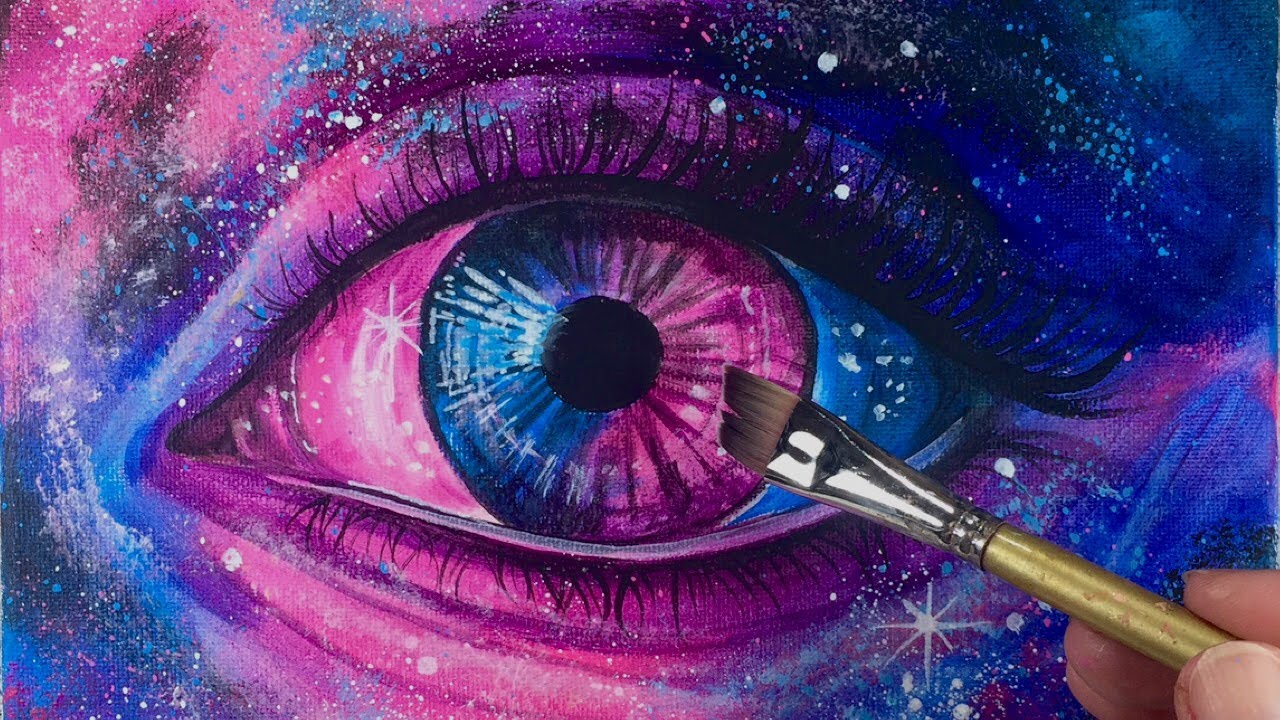In this highly detailed close-up, we see a person's delicate fingers holding a golden paintbrush with a silver tip and brown bristles, angled towards the center of the frame. The skin tone suggests the individual is Caucasian. The paintbrush is positioned over an intricate and vividly colorful painting of a human eye. The eye's iris is split into opposing hues: the left side is a deep blue, while the right side is a vibrant pink, with the central pupil rendered in solid black. Surrounding the iris, the sclera mirrors the colors in reverse, creating a striking contrast with blue on the right and pink on the left. The top and bottom eyelashes are painted lush black, adding to the eye's realistic detail. A band of purple highlights accentuate the eyebrow above and the area beneath the lower lashes. The effect is amplified by sparkling white dots scattered across the image, reminiscent of a cosmic space, blending seamlessly with the galaxy-like background of swirling purples, blues, and pinks. The top right and bottom left corners depict a dark blue sky dotted with light blue stars, while the top left corner shows a purple sky with blue stars. The intricate highlights within the eye itself add to the sense of depth and dimension in this whimsical, abstract artwork.